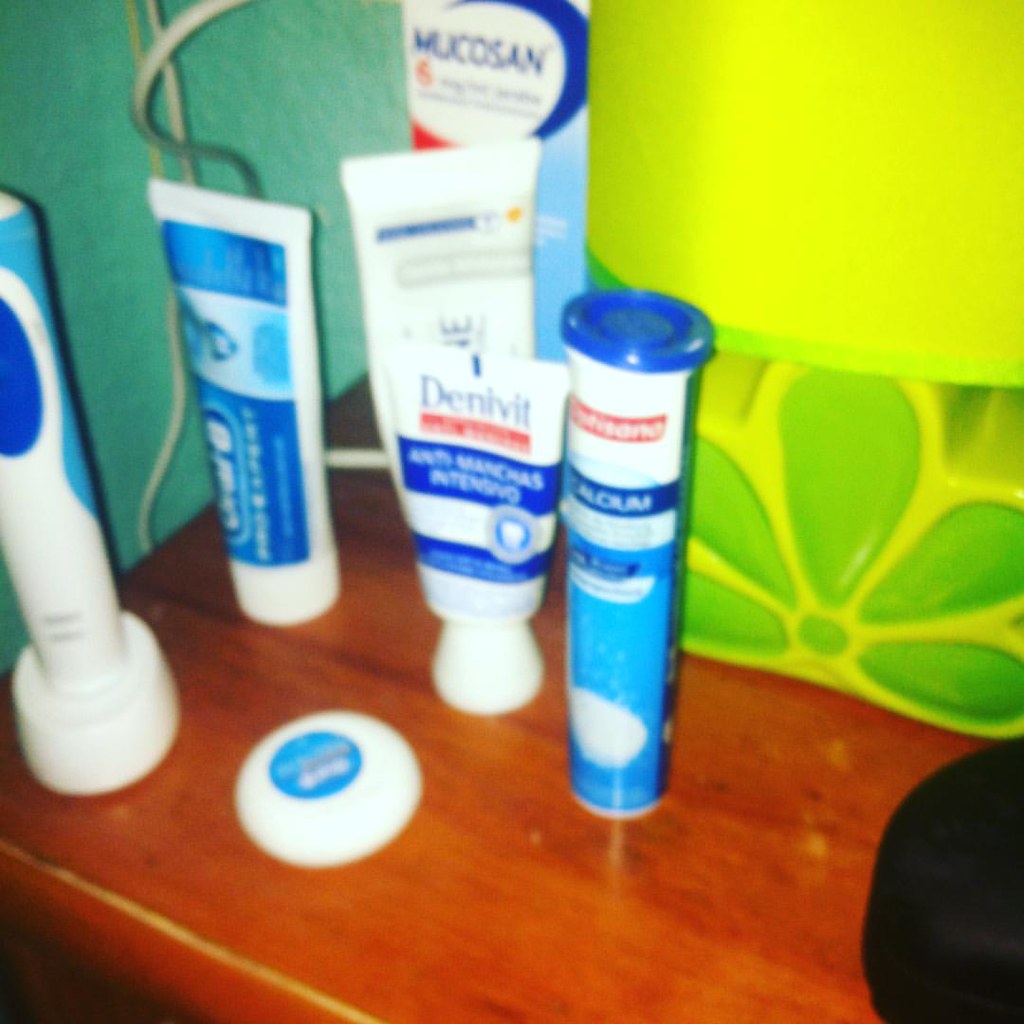The image depicts a slightly blurry, zoomed-in view of a small, rectangular, wooden nightstand table. On top of the table, there are several tubes of toothpaste, mostly blue and white, including brands like Denivit and Oral-B. In total, six toothpaste containers are visible, and their shapes and sizes vary. Toward the left side of the table, an electric toothbrush handle can be seen in its charging stand. Behind the toothpaste tubes is a green and yellow object, possibly a bag. There is also a green and lime green bucket with flower petal designs on the left side, partially cut off. Additionally, three white cable cords can be seen hanging over a green wall in the background. To the right, there's a black object partially visible in the bottom right corner, and a circular white and blue object on the bottom left corner of the table.